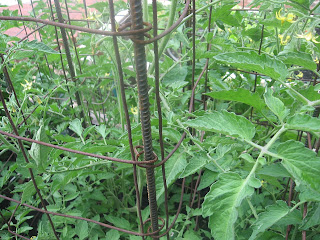This detailed image captures a close-up view of an outdoor garden, featuring a group of broad-leafed, green plants that may be tomato plants, though this is uncertain. The image shows these plants supported by a metal structure composed of iron rebar driven into the ground at the corners, forming a square framework. Twisted wire, possibly resembling chicken wire, is wrapped around the rebar at intervals of about 12 inches, creating a vertical columnar support system for the plants. The plants, which appear luscious and healthy, display yellow blossoms but no visible fruit, suggesting they are in an early growth stage. The setting seems to be part of a raised bed garden, evidenced by a visible rail and a brick sidewalk or red-tiled patio in the background. This wider-than-tall photograph focuses on the middle section of the plants and their support, cutting off before ground level but showing a small portion of the metal structure extending upwards. The scene hints at a well-maintained garden area, likely designed for efficient plant growth and care.